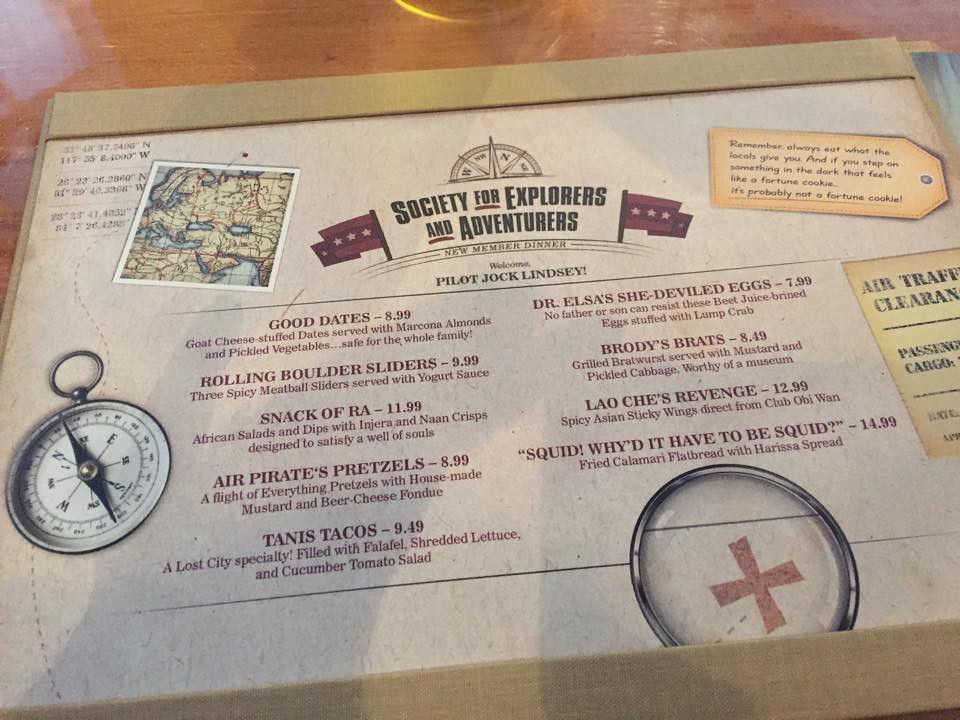The menu for the restaurant is designed to resemble an elaborate old map, yet is, in fact, a menu. At the center, it prominently displays the text: "Society for Explorers and Adventurers, New Member Dinner, Welcome Pilot Jock Lindsey." The artistic design includes thematic images such as a compass, a map, and, in the lower right corner, a magnifying glass that appears to illuminate a steel cross. 

The menu features a variety of creatively named dishes:
- Snack of RA
- Air Pirates Pretzels
- Tannis Tacos
- Brody's Brats
- Lao Che's Revenge, which humorously adds, "Squid, why did it have to be so squid?"

This unique and intricately designed menu enhances the dining experience by immersing guests in a sense of adventure, perfectly fitting the restaurant's theme.